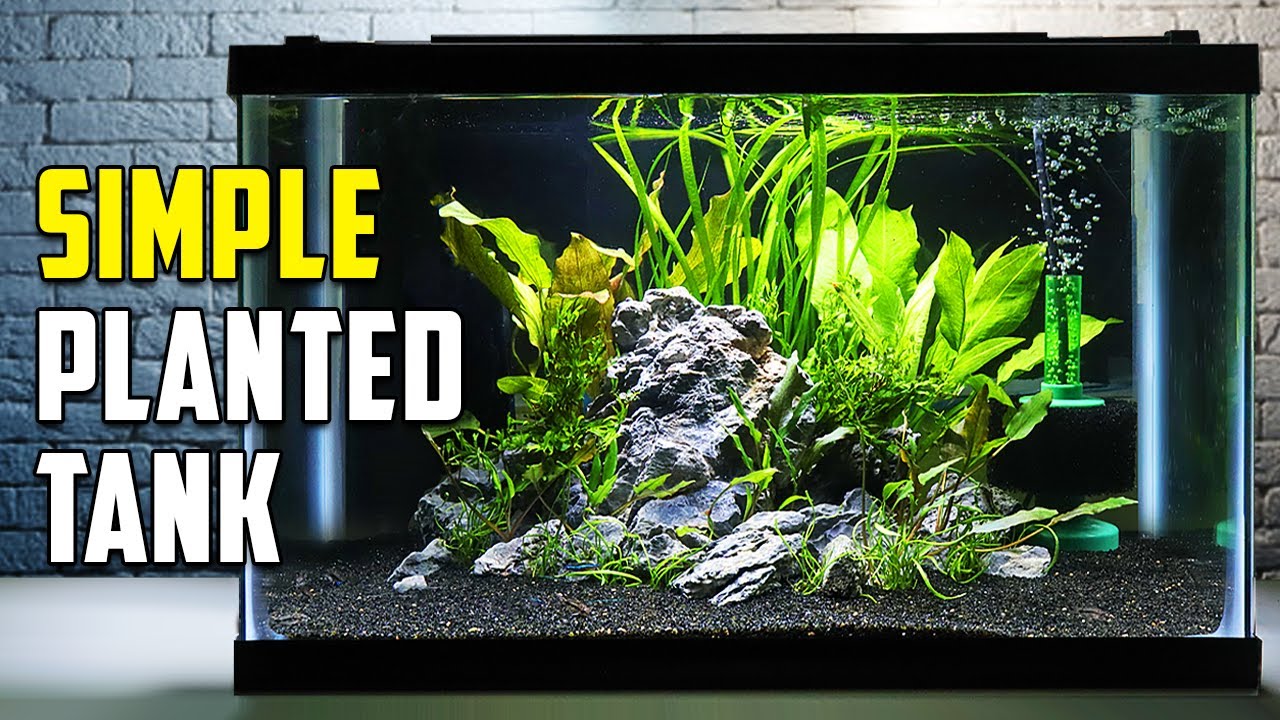The image depicts a clean and detailed rectangular fish tank, most likely used for aquatic plants rather than fish. Positioned on a table, the tank is set against a white-painted brick wall backdrop. The tank itself features a black top and contains an assortment of underwater plants, meticulously arranged with a variety of rocks at the base—some white, some colored, with textures ranging from smooth to craggy. Prominently displayed in the tank are two large leafed plants on either side of the arrangement. It also houses a water filter in the back, producing bubbles that rise and spread horizontally at the surface. Inside, the substrate is composed of sand. Notably, the tank bears a promotional design with the words "simple" in yellow and "planted tank" in white, typical of a YouTube thumbnail style, indicating it could be an advertisement or a video still.